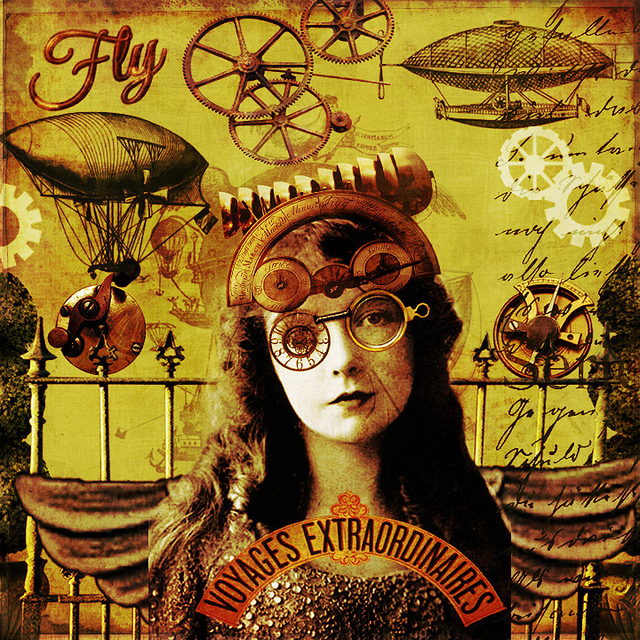In the center of this sepia-toned digital artwork is the upper body of a woman with long dark hair, tilting her head slightly to the left, staring directly at the viewer. Her face is adorned with unique glasses; the lens on her left eye resembles a clock while the right lens transforms into a compass-like design. Resting on her forehead is another pair of glasses, incorporating navigational instruments. She wears a metallic hairband, detailed with gold and red accents and an inscription. Below her, the words "Voyages Extraordinaires" are elegantly displayed in a semi-circle.

The background contributes significantly to the steampunk aesthetic, filled with an assortment of gears, prototype flying machines, hot air balloons, and blimps with intricate designs, some featuring human-powered mechanisms. There is a decorative metal fence behind her, with wing-like structures hanging beside her. In the top left corner, the word "fly" is prominently written in red cursive lettering, while elegant cursive script stretches from top to bottom on the right side of the image. The entire scene exudes a vintage and adventurous atmosphere, blending the fantastical elements of steampunk with detailed mechanical artistry.